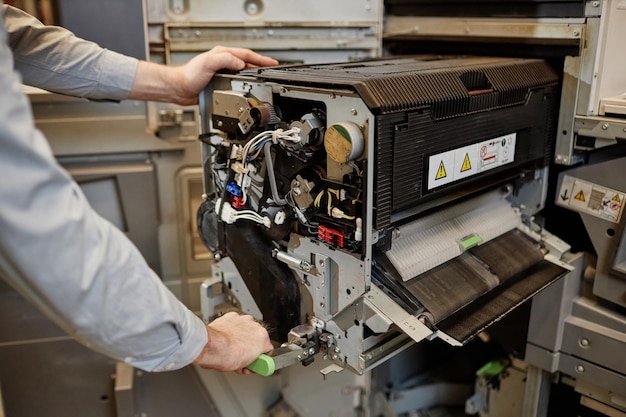The image captures a man wearing a light gray long-sleeved shirt, with only his arms and hands visible, working on a large piece of machinery situated on the left-hand side. His left hand rests on the top of the machine, and his right hand grasps a green handle at the lower part of the machine. The machine, likely an old industrial printer or copier, has its side panel removed, exposing its internal mechanisms including numerous wires in red, white, and blue. The front of the machine features a set of warning labels with yellow triangles on a white rectangular background. Furthermore, there's an opening below the labels that suggests it might be the exit point for printed or produced materials. The machine appears to have a mix of black and gray components, with some brown elements where paper or other materials might be fed through. Surrounding the main subject, other industrial-looking machines are visible in a setting that seems to be a workshop or an unfinished room, adding to the industrious atmosphere of the scene.